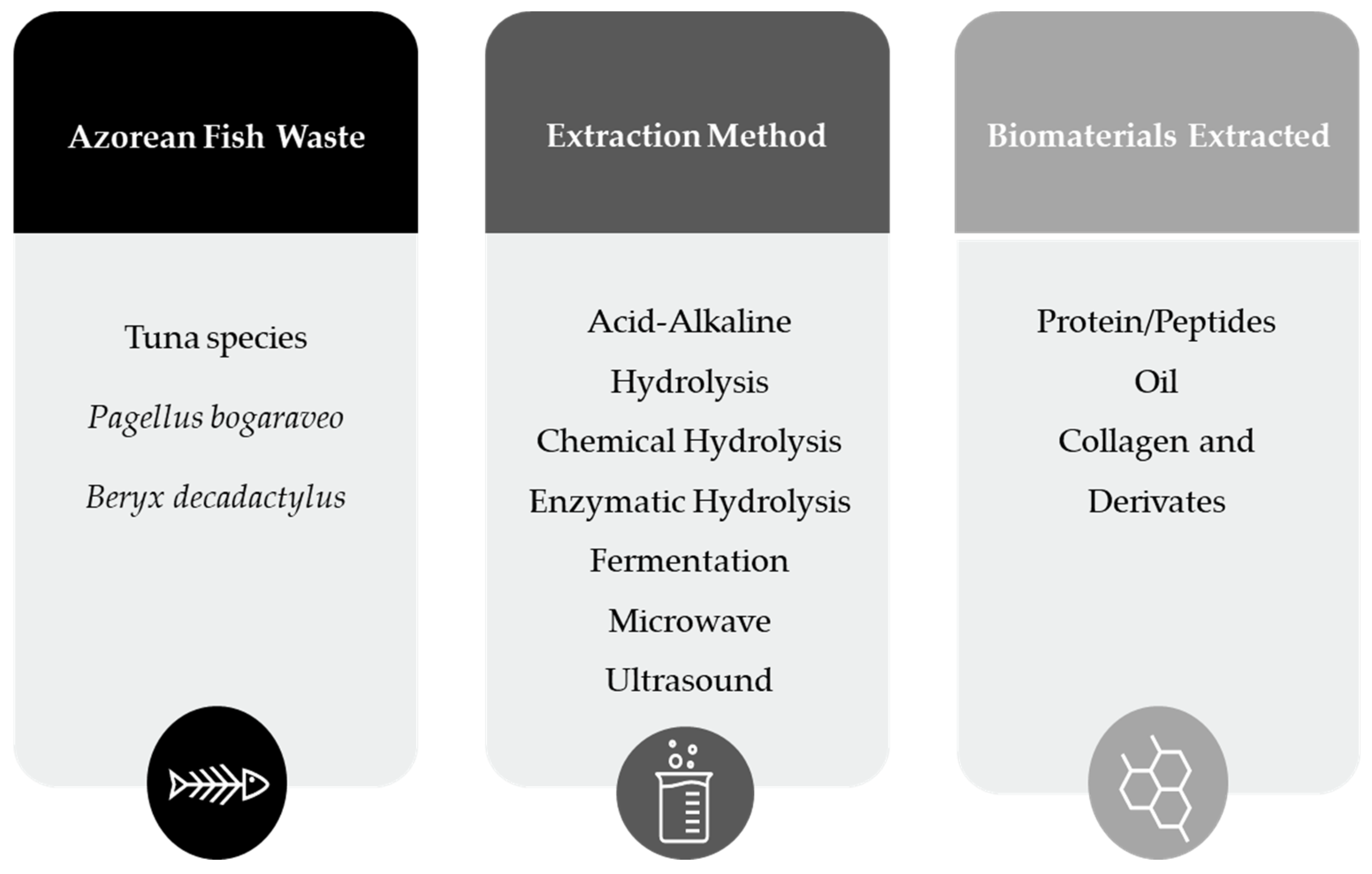The image is an informative infographic featuring three vertical, rounded rectangular sections, each in different colors. The leftmost section is predominantly black with a central white area containing black text. This section is headlined "Azorean Fish Waste" and lists "Tuna species, Paguelis balgorivale, and Beryx decaductilis". A small illustration at the bottom displays a stick figure of fish and bones. The middle section transitions to a dark gray color, also with a central white area containing black text. This section is titled "Extraction Method," and enumerates various methods: "acid alkaline, hydrolysis, chemical hydrolysis, enzymatic hydrolysis, fermentation, microwave, and ultrasound". An illustration at the bottom features a beaker with water and bubbles. The rightmost section is light gray at the top and bottom with a white center, headlined "Biomaterials Extracted". It lists "protein/peptides, oil, collagen, and derivatives". At the bottom, there's an illustration showing the organic chemistry structure of the extracted biomaterials.